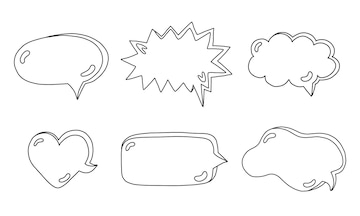The image showcases six distinct speech bubble outlines set against a white background, reminiscent of those found in comic strips or cartoons. Arranged in two rows of three, each bubble features unique shapes and styles rendered in sleek black outlines with shiny highlights. In the top row, the first bubble is an oval shape with two small bean shapes inside it. The second is a spiky, cloud-like burst, typically used for exciting or loud expressions. The third bubble is shaped like a fluffy cumulus cloud. In the bottom row, the first bubble is in the shape of a heart. The second bubble is a rectangular shape with rounded corners, and the final bubble has an irregular, amoeba-like shape. The overall design evokes a sense of playful communication, similar to sticky notes or Post-Its.